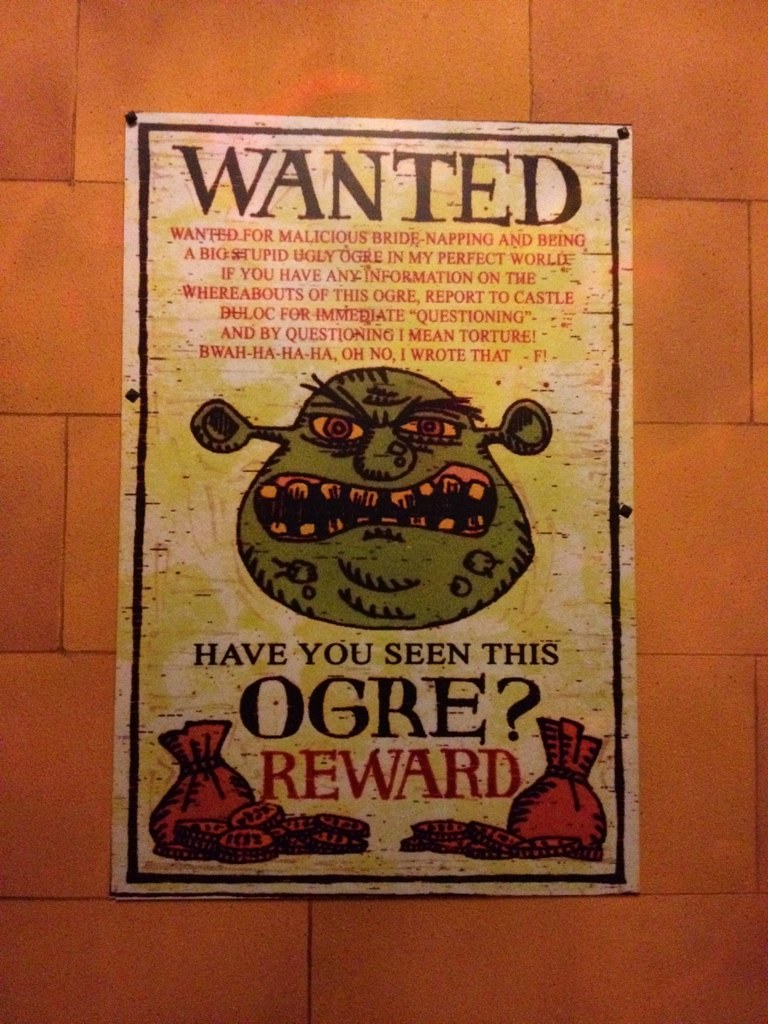The image depicts a colorful, cartoonish "Wanted" poster tacked onto a textured, orange-reddish wall that resembles large bricks with a faux stone finish. The poster, set against a predominantly white background with dark green splotches and outlined in a black border, urgently seeks information about an ogre. Bold, brown letters at the top exclaim "WANTED," and below, in red text, the poster details: "Wanted for malicious bride-napping and being a big stupid ugly ogre in my perfect world. If you have any information on the whereabouts of this ogre, report to Castle Duloc for immediate questioning, and by questioning, I mean torture. Bwa ha ha ha. Oh no, I wrote that." The centerpiece of the poster is a caricature of an ogre that resembles Shrek, featuring a large green face with warts, rotted yellow teeth, and odd ears that stick out. The ogre’s mean yellow and green eyes glare out from the poster. Below the ogre's face, red text asks, "Have you seen this ogre?" followed by "REWARD," flanked by images of red money bags and coins. The vibrant colors used on the poster include black, white, red, green, yellow, and various shades of brown, adding to its eye-catching, cartoonish style.